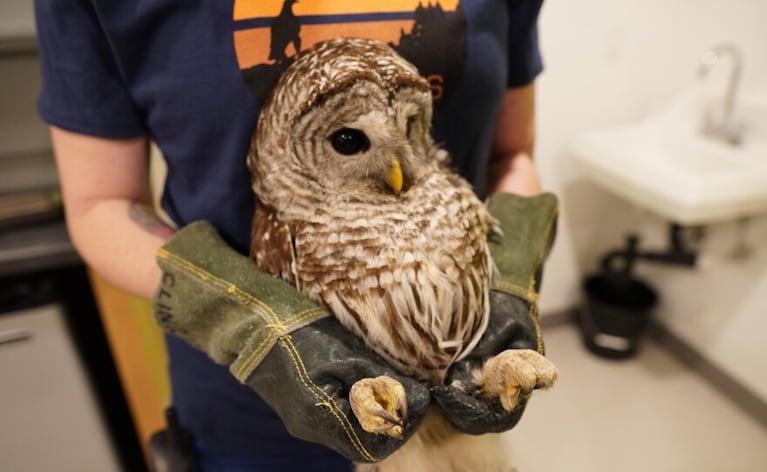The photograph captures a detailed, well-lit close-up of a woman holding an owl. The owl, prominently centered in the image, boasts a feather coat in shades of cream and light brown. Its round black eyes gaze off to the right, above a sharp yellow beak. The woman, whose upper body is mostly cropped out above the chest, holds the owl securely by its lightly yellow feet with her arms, adorned in sturdy gloves that range from light to dark green with yellow stitching for added durability. She wears a dark blue shirt featuring a partially obscured circular logo in orange, dark blue, and black. The woman appears Caucasian, judging by the visible skin on her arms. The bright, clear setting highlights the subject, leaving the background blurry except for noticeable elements—a white and silver faucet to the right with a black bucket below. The image’s composition and clarity emphasize the owl and its handler as the focal points.